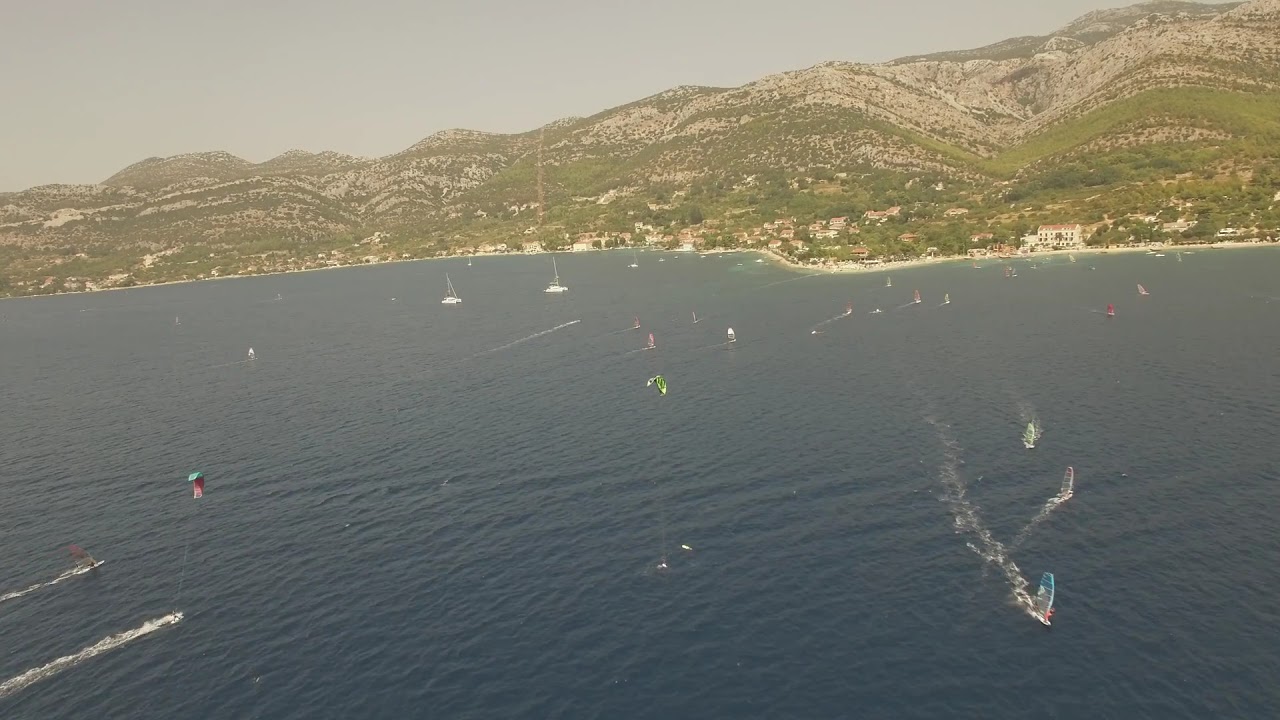This photograph, taken from an elevated perspective—likely a plane or drone—captures a sprawling daytime view of a large lake with a mountainous backdrop. Despite the image not being of the highest quality, a brownish-gray haze or smog permeates the scene, casting a muted overcast over the entire landscape. The deep blue water in the foreground, somewhat tainted by the brown haze, remains relatively calm, featuring subtle ripples. Numerous boats populate the lake: motorboats leave distinct white wakes, some appearing to tow kites, while sailboats gliding gracefully through the water. Additionally, jet skis sporadically cut through the surface, and there are visible instances of people engaging in parasailing.

The distant shoreline is thin and narrow, giving way to a majestic range of rounded, lightly sanded mountains interspersed with rows of moss-green foliage. Contrasting with the activity on the water, the upper portion of the image transitions to a dark gray and brown sky, heavily shrouded in thick haze. Buildings are discernible on the land, adding to the complexity and vibrancy of the scene, while the bottom two-thirds of the image focuses predominantly on the lake, where diverse water activities dominate, highlighting a lively yet serene aquatic landscape.